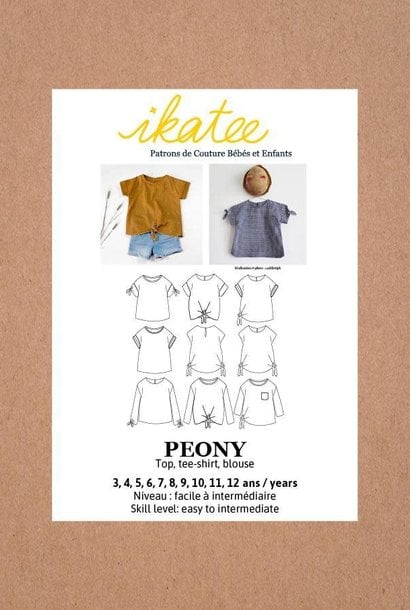The image is an advertisement for infant clothing, presented on a white poster framed by a brown-beige border. At the top of the white section, the brand name "Ikatee" is written in yellow cursive. Below the brand name, the text reads "Patron's Day, Kostura, Baby, Infante," indicating a focus on baby fashion. The top portion of the ad features two color images: on the left, a brown t-shirt paired with blue denim shorts, resembling Daisy Dukes; on the right, a dark gray or purplish short-sleeve shirt with possible ribbons or bows, displayed on a stylized head or hanger. 

Beneath these images, there are three rows of black-and-white line drawings showcasing various styles of tops, which include t-shirts and blouses. Each row contains three different designs, suitable for children aged 3 through 12 years. The word "Peony" is prominently printed under these drawings, followed by descriptions of sizes and skill levels for making them, such as "Nouveau," "Facilité," "Intermediaire," indicating that the designs are easy to intermediate in difficulty.